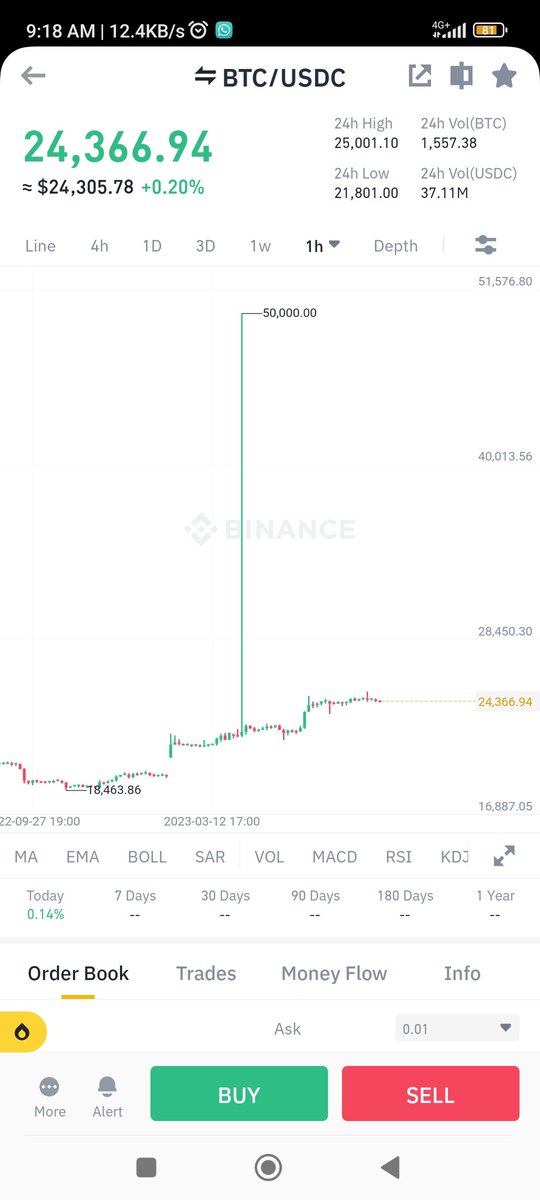This screenshot captures a trading app interface, focused on the Bitcoin to US Dollar (BTC/USD) trading page. The screen has a white background with a subtle finance watermark. The central portion of the screen prominently features a detailed graph showcasing Bitcoin's performance over time.

In the top left corner, the current Bitcoin value is displayed in green at $24,366.94, indicating a 0.2% increase for the day. Next to this, there are quick statistics showing the 24-hour high, low, volume, and other relevant metrics for BTC/USD.

The interface includes various navigation and functional buttons:
- Top left: A back button.
- Top right: Buttons for sharing, favoriting, and modifying the graph display settings.

Additionally, across the top of the phone screen, you'll see standard indicators such as battery life, signal strength, the current time, data speed, an alarm icon, and a WhatsApp icon.

Below the graph, there are multiple selectable time frames for viewing Bitcoin’s performance, including options for 1 hour, 4 hours, 1 day, 3 days, 1 week, and more, along with buttons for depth settings and line options.

At the very bottom of the screen, there are buy and sell buttons, along with an order book for managing asks and placing orders. The section just beneath the graph includes timestamps and value markers to help users analyze the data more effectively.